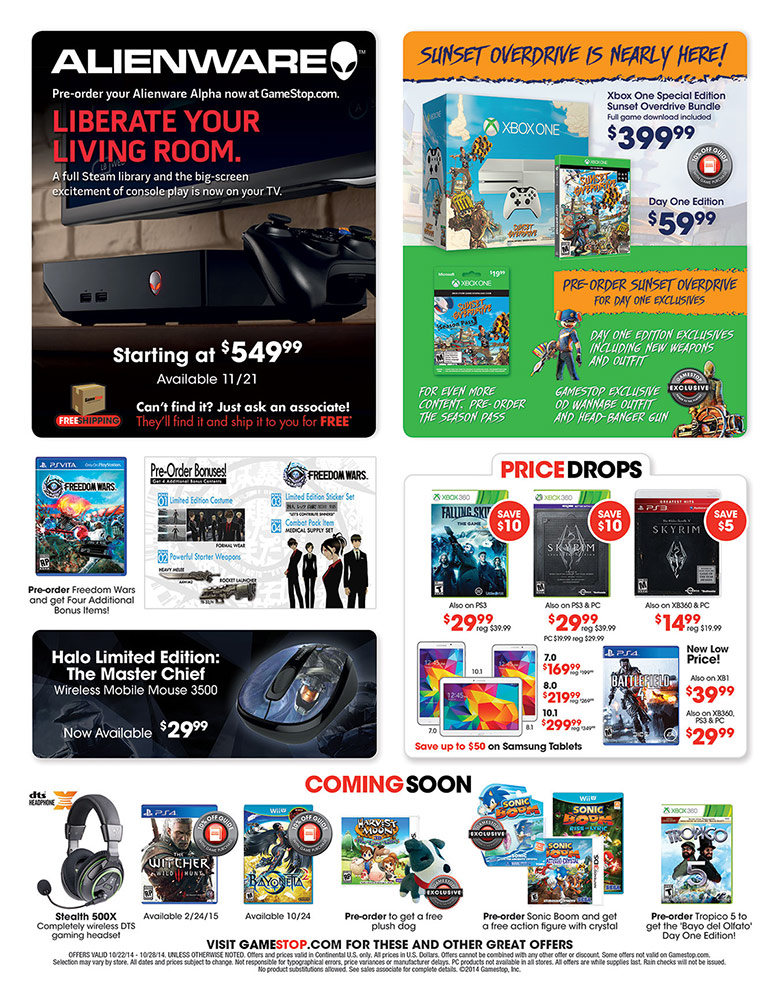This image is a digital version of a circular advertisement from GameStop. The layout has four distinct quadrants at the top with an additional horizontal section along the bottom. 

In the upper left quadrant, there's an ad for Alienware featuring a sleek gaming system set beneath a flat-screen TV. A black remote control leans against the system. The ad highlights that prices start at $549.99 and notes availability from 11-21.

The upper right quadrant focuses on the game "Sunset Overdrive." The text reads, "Sunset Overdrive is nearly here." Beneath it, there's an Xbox bundle for "Sunset Overdrive" priced at $399.99 and the individual game available for $59.99.

In the lower left quadrant of the second row, there’s an advertisement for the "Halo Limited Edition Master Chief Wireless Mobile Mouse" priced at $29.99. Adjacent to it is a pre-order ad for "Freedom Wars."

The lower right quadrant showcases a sales section featuring price drops for various games. The horizontal bottom section also highlights additional deals and promotions, completing the detailed advertisement layout from GameStop.